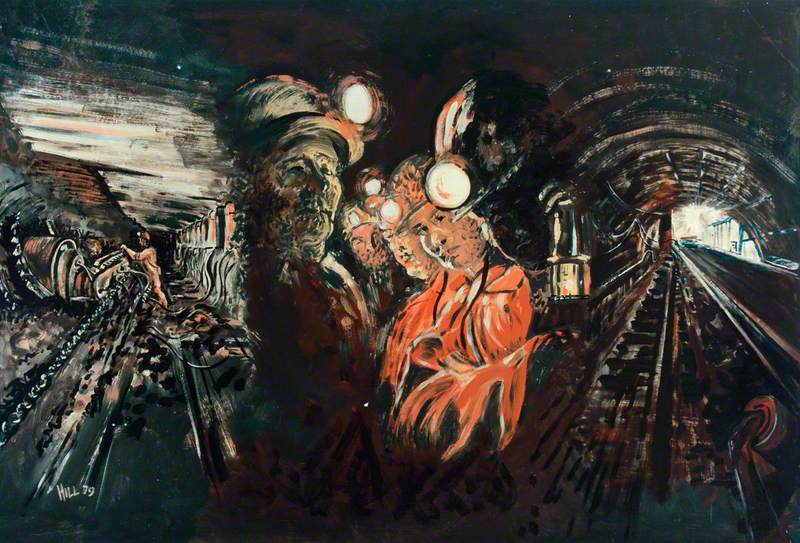This detailed painting illustrates a dark, ominous scene inside a coal mine. The image is primarily black, with muted lighting creating an eerie effect. On the far right, there's an arched tunnel with train tracks running through it, where a dim light can be seen at the end. Moving towards the center, four coal miners are prominently depicted, their faces and shoulders illuminated by headlamps attached to their hard hats. Their expressions are indistinct, yet it's clear they are staring straight ahead, as if facing a camera. One of the miners stands out in an orange jumpsuit. To the far left, another tunnel with a flat roof is visible. Within this tunnel, a lone worker is seen, appearing to be engaged in some task, possibly leaning on something. Overall, the painting powerfully conveys the harsh, shadowy environment of the mining world, with a focus on the miners' resilience and solidarity in the face of adversity.